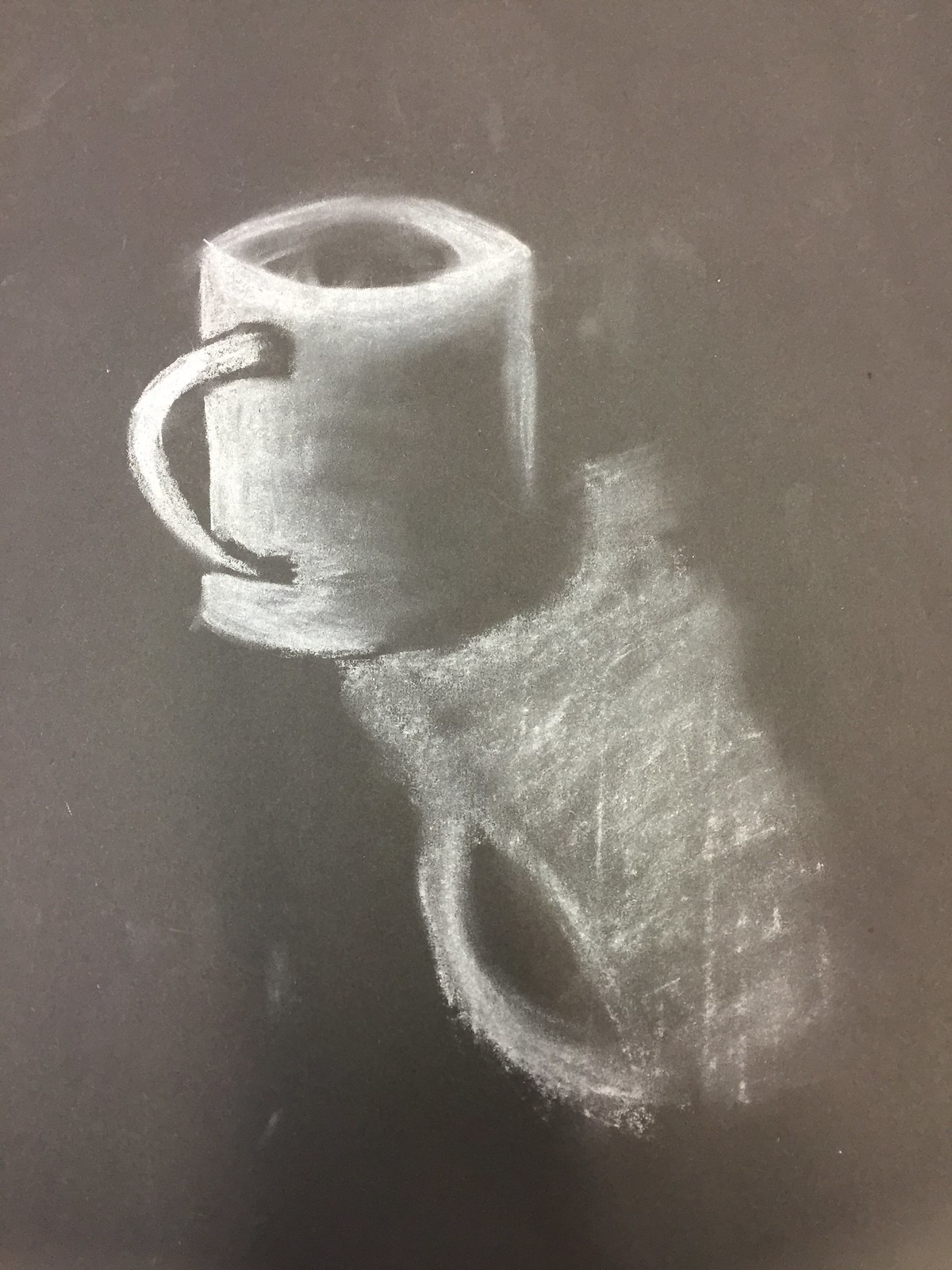In front of me is an intriguing painting depicted with meticulous detail. The centerpiece is a tea mug, rendered in varying shades of white that capture the subtleties of light and shadow. A crisp black outline enhances the realism, highlighting the reflective properties of the mug. The background is a deep, uniform black, which starkly contrasts with the mug, making it stand out prominently. To the right of the mug, there is a nuanced reflection, displaying an array of lighter shades that suggest a light source off to the side. The reflection is irregularly shaped yet discernibly captures the contours of the mug and its handle. This juxtaposition of light and dark, along with the intricately detailed reflection, makes for a remarkably beautiful and thought-provoking painting.